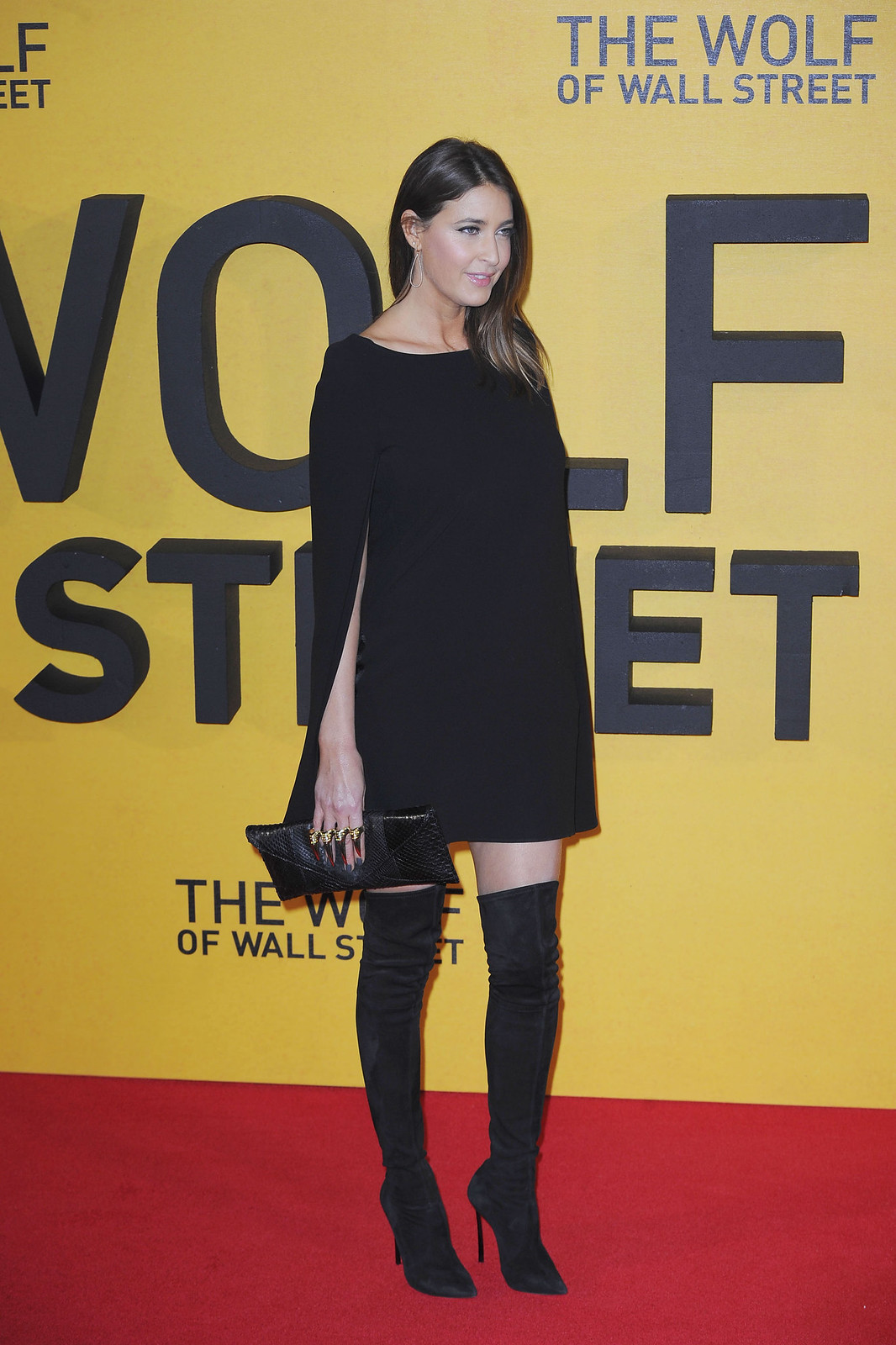This photograph captures a fashionably dressed woman standing indoors on a red carpet. The central focus of the image is the woman, who appears slightly off-center and is looking to her right, away from the camera. She is wearing a black cape top paired with high black boots that reach just above her knees. She accessorizes her ensemble with a black clutch in her right hand and rings on her fingers. The backdrop features a wall adorned with the words "The Wolf of Wall Street" repeated multiple times in large, bold black letters. The wall itself is yellow, adding a striking contrast to the scene. The overall color scheme in the image includes red, black, yellow, tan, and gold, indicating a vibrant setting, possibly at a movie premiere or special event. The setting suggests an indoor location without a clear indication of the time of day.